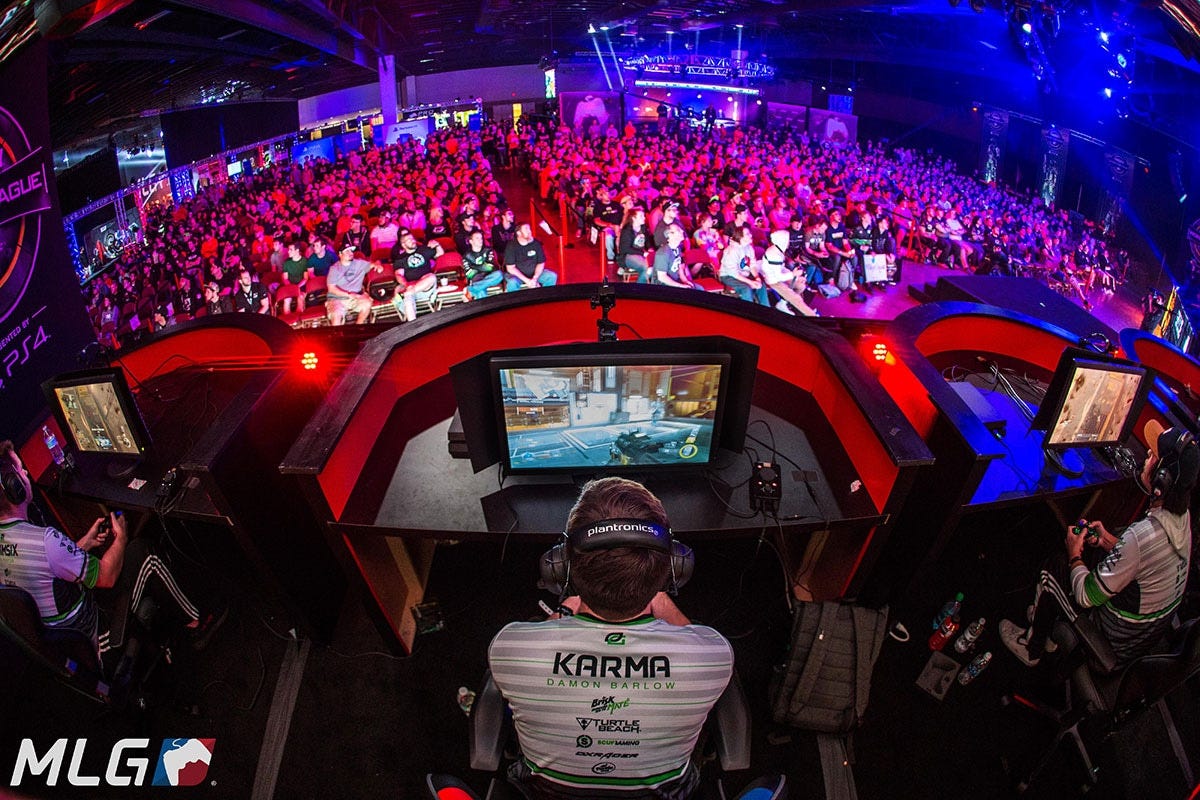A high-angle shot captures an exhilarating live event, prominently branded with the MLG (Major League Gaming) logo in the corner. Three individuals are stationed in separate booths, each equipped with a screen and a controller. The central player, identified by the name "Karma" on his white shirt with gray stripes, is immersed in the game, adorned with headphones and flanked by a webcam. The players on either side are dressed in matching attire, distinguished by green bands on their sleeves and a green neckline. The booths are designed for focus and separation, featuring vivid red interiors with black counters. Extending into the expansive crowd, a sea of spectators fills the venue, illuminated by dynamic lighting that bathes the audience in hues of blue, purplish-pink, and yellow. The front rows of the crowd are particularly vibrant, highlighted by brighter, yellowish lighting, enhancing the electrifying atmosphere of the event.